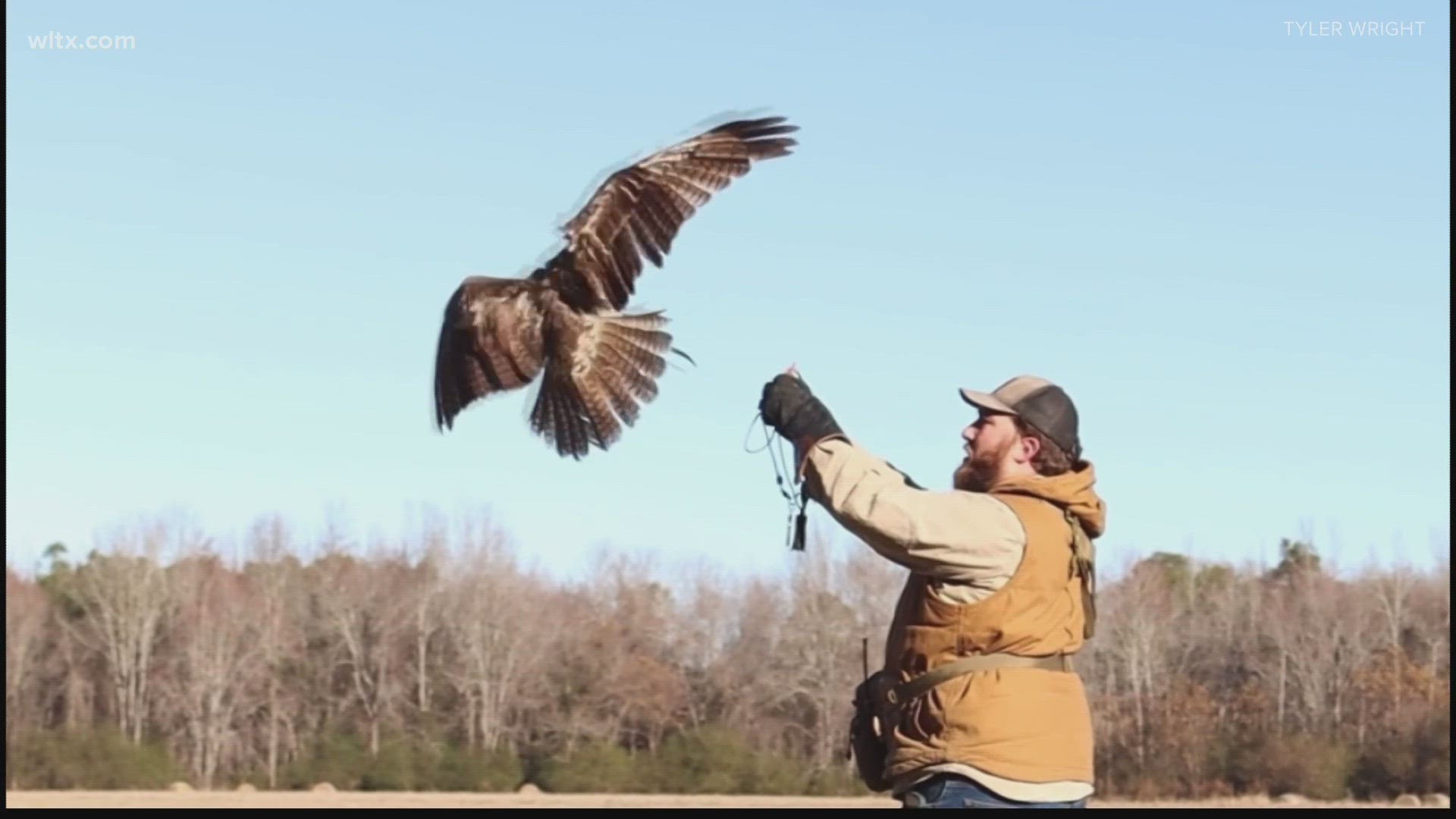In this outdoor daytime color photograph, there is a white, slightly heavyset, bearded man with brown hair in the foreground. He is wearing a baseball cap, black gloves, a tan jacket, a light brown vest, a beige long-sleeve shirt, and blue jeans. The man is standing in profile, facing the left side of the frame, with his left arm fully extended. He is engaged in a bird training activity, either releasing or receiving a bird of prey. The bird, which could be a hawk, eagle, or falcon, is slightly above and to the left of the man with its wings fully extended, tail feathers fanned out, and its back facing the camera. The bird, which has a brown and white plumage, appears to be in mid-flight. The background features a cloudless, sunny sky and a line of wooded trees that are barren of leaves, indicating it might be late fall. There are some shrubs on the ground as well. The top of the image features white text that reads "wltx.com."